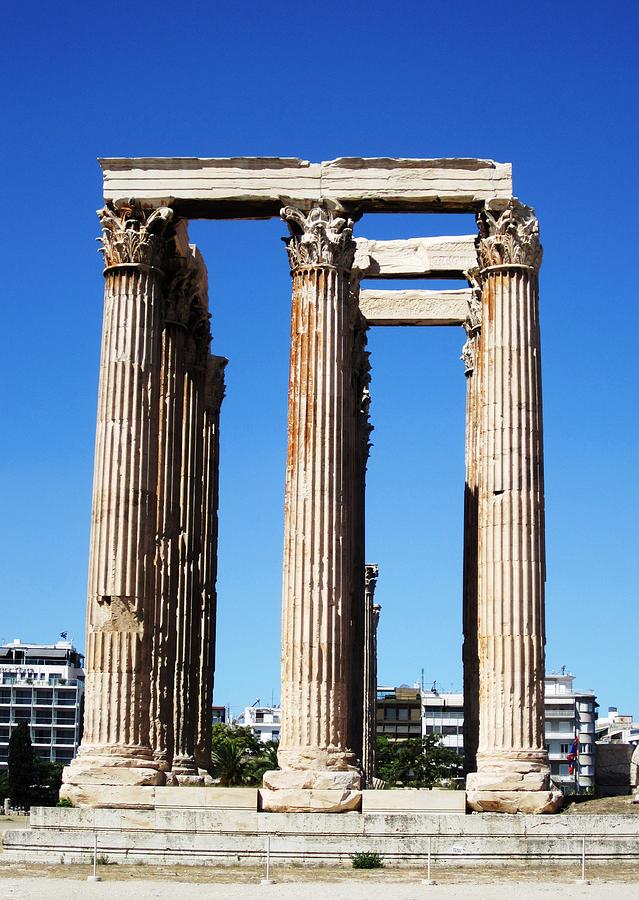The photograph showcases an impressive display of ancient ruins, featuring a series of classical columns set against a deep blue sky that transitions from a darker shade at the top to a lighter hue near the horizon. Central to the image are three prominent columns that rise from a stone platform with three to four steps leading up to them. These columns, displaying the characteristic beige color typical of ancient architecture, extend vertically with fluted ridges and decorative capitals. Behind these primary columns, rows of additional columns stretch into the distance, giving a sense of depth and scale.

In the background, modern six-story white buildings and a few flags on the bottom right corner provide a stark contrast to the ancient scene. Horizontal stone lintels rest atop some of the vertical columns, particularly noticeable on the front row and a few in the middle and right rows. This architectural assembly suggests remnants of a once-grand structure, possibly of Greco-Roman origin, now standing as a testament to historical grandeur. The clean, clear sky further enhances the visual prominence of the ruins against the urban landscape.